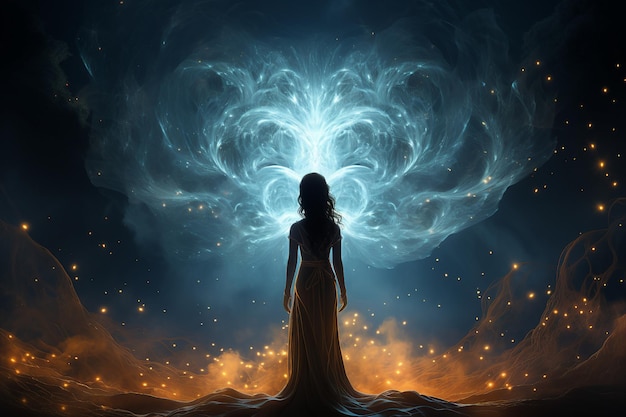The image depicts a woman in a surrealistic, intergalactic scene that combines elements of digital art and AI-generated imagery. The woman stands with her back towards us, her arms hanging by her sides, emphasizing her slender figure. She wears a long, flowing dress, with an extended train that contrasts with the tightly fitted bodice, highlighting the curve of her waist. Her wavy, dark hair cascades down her back and seems to be blowing gently off her shoulders.

She faces an ethereal sky filled with dynamic patterns. The upper part of the sky features swirling blue and white wisps that resemble clouds or smoke, while the lower part transitions into vibrant golden and orange hues, dotted with small lights or embers that give the illusion of floating fireflies. This light play enhances the mystical atmosphere. Below her feet, the ground appears molten and wavy, contributing to the otherworldly setting. The intricate combination of celestial and fiery elements around the woman creates a striking contrast, making the scene appear both mesmerizing and haunting.